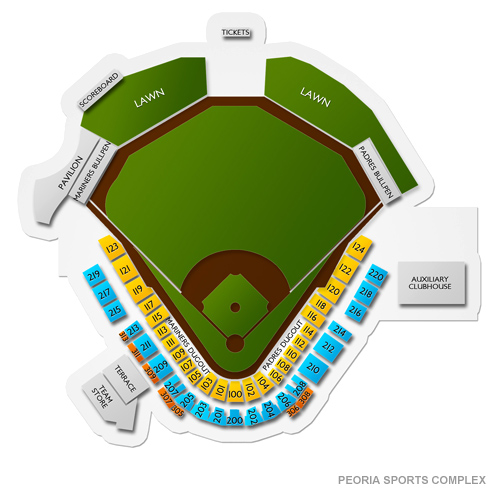This detailed seating map of the Peoria Sports Complex is displayed from an overhead perspective. In the bottom-right corner, the map is labeled "Peoria Sports Complex." The image primarily features a green area representing the baseball diamond, complete with field lines. At the top of the map, there's a section resembling an upside-down pyramid, which includes various labeled areas such as the Pavilion, Mariners Bullpen, Scoreboard, Lawn, Tickets, and Padres Bullpen.

Surrounding the diamond, there's an inner curved section with yellow seats, followed by an outer curved section showcasing blue seats. Additional marked areas include the Terrace, Team Store, and Auxiliary Clubhouse. The map is a schematic representation with no photographic elements and includes no people, animals, plants, vehicles, or aircraft.